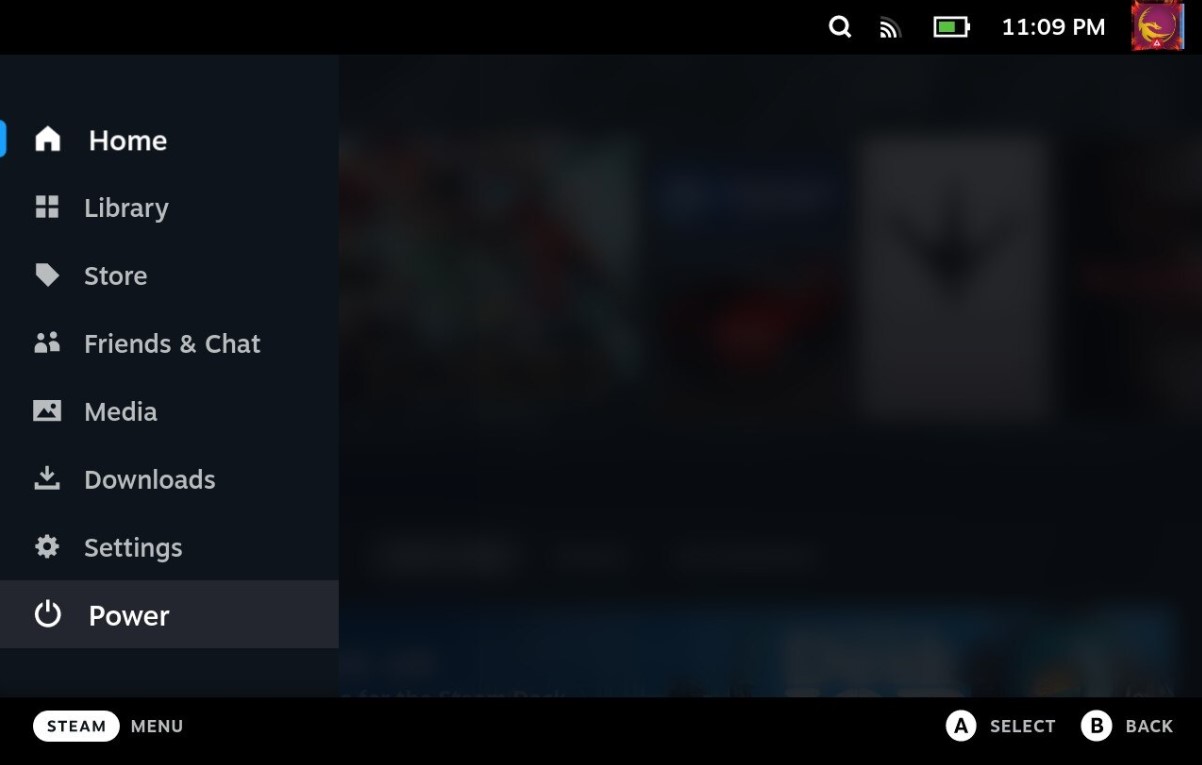The image features a user interface with a primarily black border at the top and bottom. At the top, there are several icons, including a magnifying glass, a Wi-Fi symbol, and a battery indicator showing roughly two-thirds capacity. The time displayed is either 11:09 PM or 11:09 AM, to the right of which is an intricate design incorporating gold, purple, red, and blue colors.

The central portion of the image contains a blurry visual element that appears to display titles or thumbnails of movies, although the specifics are unclear due to the blur.

Along the left side of the interface is a vertical menu with several options, each accompanied by a representative icon. The menu options are as follows:

1. Home
2. Library
3. Store
4. Friends and Chat
5. Media
6. Downloads
7. Settings (represented by a gear icon)
8. Power

Towards the bottom, in an otherwise blank area, the phrase "Theme Menu" is written. On the right side, there are prompts indicating that pressing 'A' will select an option, while pressing 'B' will take the user back.